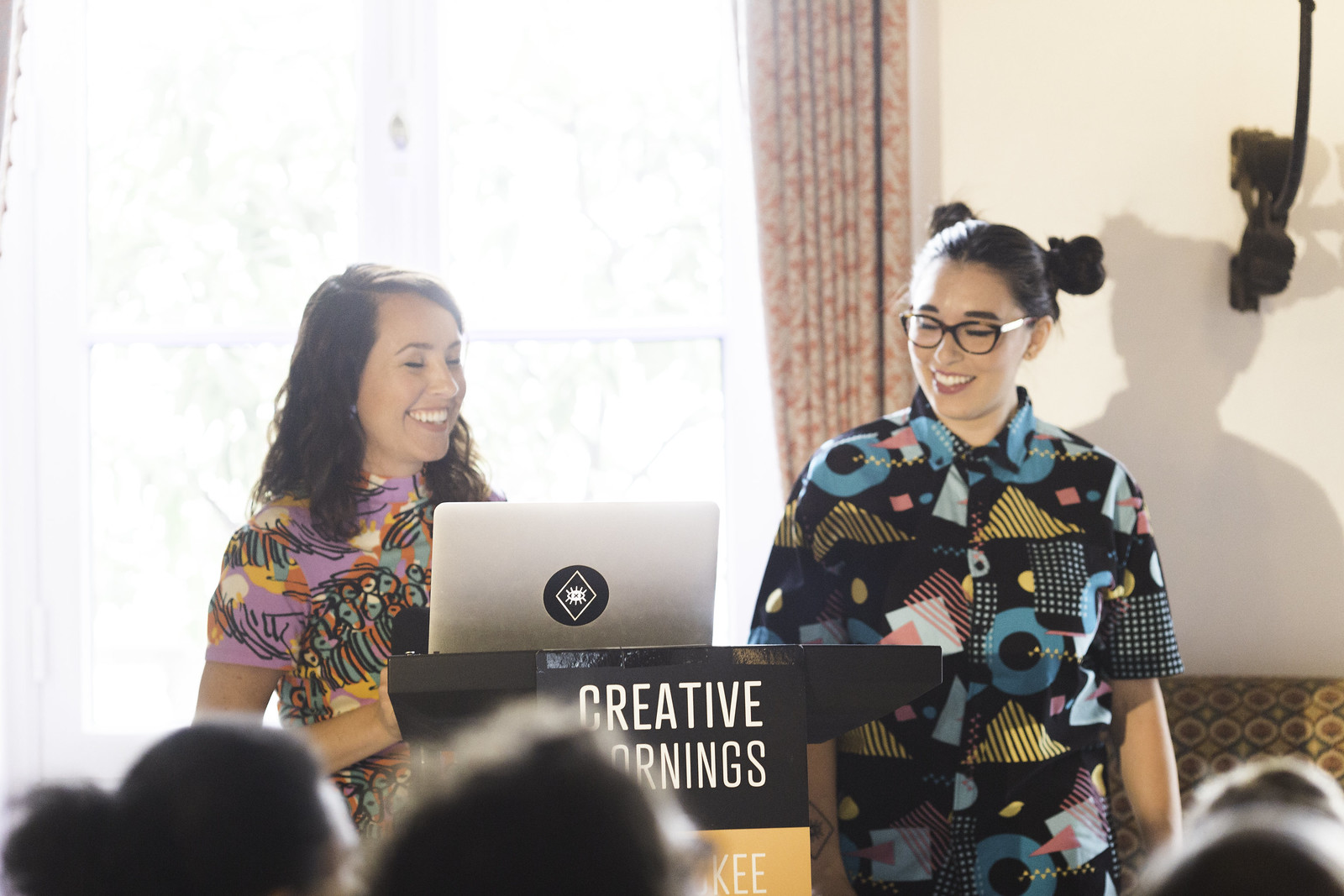In this color photograph, two women are standing at a black podium adorned with a sign that reads "Creative Mornings" in white lettering, with an unreadable orange sign with white print below it. Both women are smiling and engaged in conversation as they look at a laptop decorated with a black-and-white sticker.

The woman on the right has brown hair styled in pigtail bunches and wears glasses. She is dressed in an abstract t-shirt featuring shapes like circles and stripes in colors including black, blue, light blue, and pink. The woman on the left has long brown hair flowing down and is wearing a vibrant, multicolored top patterned with black squiggly lines and shades of purple, yellow, blue, and red.

Behind them is a bright window framed by dark pink and white curtains, and a beige wall is visible to the right. A small crowd is watching them with anticipation, with several heads visible in the foreground. The scene conveys a sense of creativity and engagement, underscored by the dynamic colors and attentive audience.